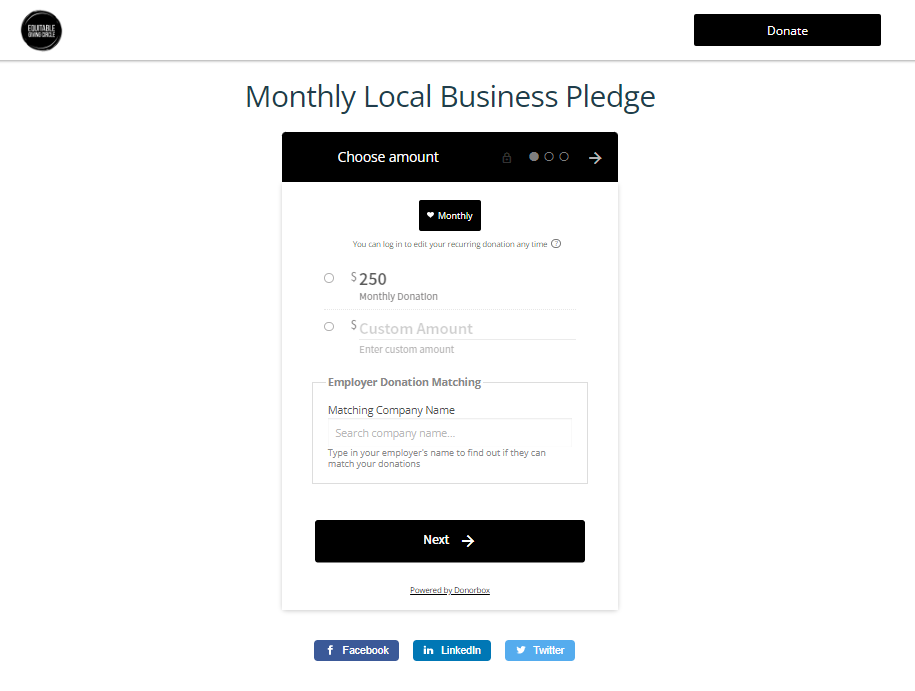This image depicts a webpage designed for pledging monthly donations to a business. 

At the top left of the page, there is a blurry logo, making the text inside it indistinguishable. To its right, a prominent black rectangle with the word "Donate" written in white stands out. The main heading in bold, "Monthly Local Business Pledge," is central to the page. Below this heading, the section "Choose Amount" is introduced, accompanied by a small gray lock symbol, signifying security. Adjacent to this are three circles outlined in gray, with only the first one filled in. A gray arrow pointing to the right is aligned with these circles.

On a white background, the word "Monthly" is displayed inside a black rectangle with a small white heart embedded in it. Beneath this section, the text reassures users that they can log in anytime to edit their recurring donation. 

The donation options include:
1. A $250 monthly donation option with an unticked gray-outlined circle to its left.
2. A customizable donation option, which includes a circle to its left (also not selected) and light gray text reading "Custom Amount" with an additional field labeled "Enter Custom Amount" beneath it.

Below these options, there's a section for "Employer Donation Matching" with a box where users can input their company name. Instructions in light gray instruct users to "Search Company Name" to discover if their employer can match their donations.

At the bottom of the page, there's a notable long black rectangle with the word "Next" in white, accompanied by a white arrow pointing right. Right below it, the site indicates it is "Powered by Donor Box," underlined in black. The very bottom of the page features three social media icons: Facebook on the left, LinkedIn in the center, and Twitter on the right.

The overall design emphasizes the ease of setting up recurring donations and offers additional features such as employer donation matching.